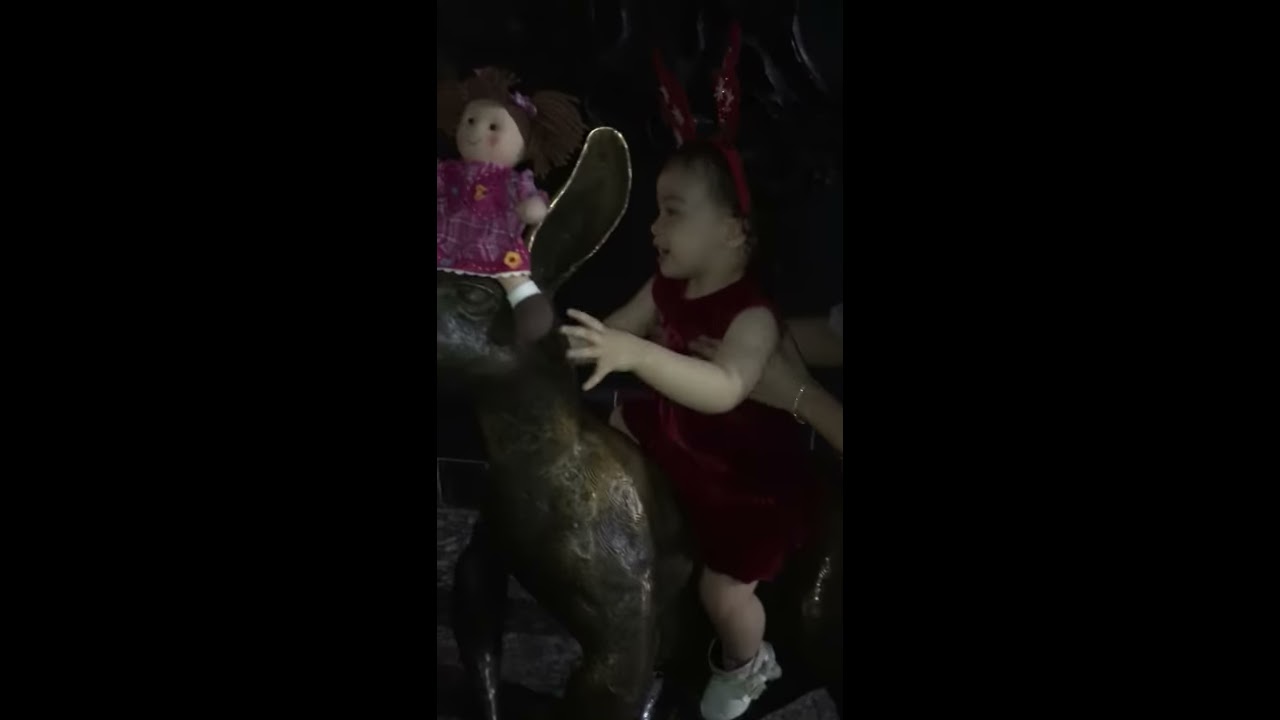In an indoor scene captured vertically with letterboxing on both sides, a young girl, around two years old, is the central subject. She’s seated on a dark-colored ceramic rabbit and is wearing a dark red sleeveless dress along with white shoes. Her head is adorned with a red band. An adult, identifiable by a gold bracelet on her left wrist, is holding the girl steady by her armpits. The girl has placed a pink-dressed doll with brown hair and a pink ribbon on the rabbit's head. The blurred and dark background makes the figures stand out distinctly, adding to the intimate and tender moment being captured.